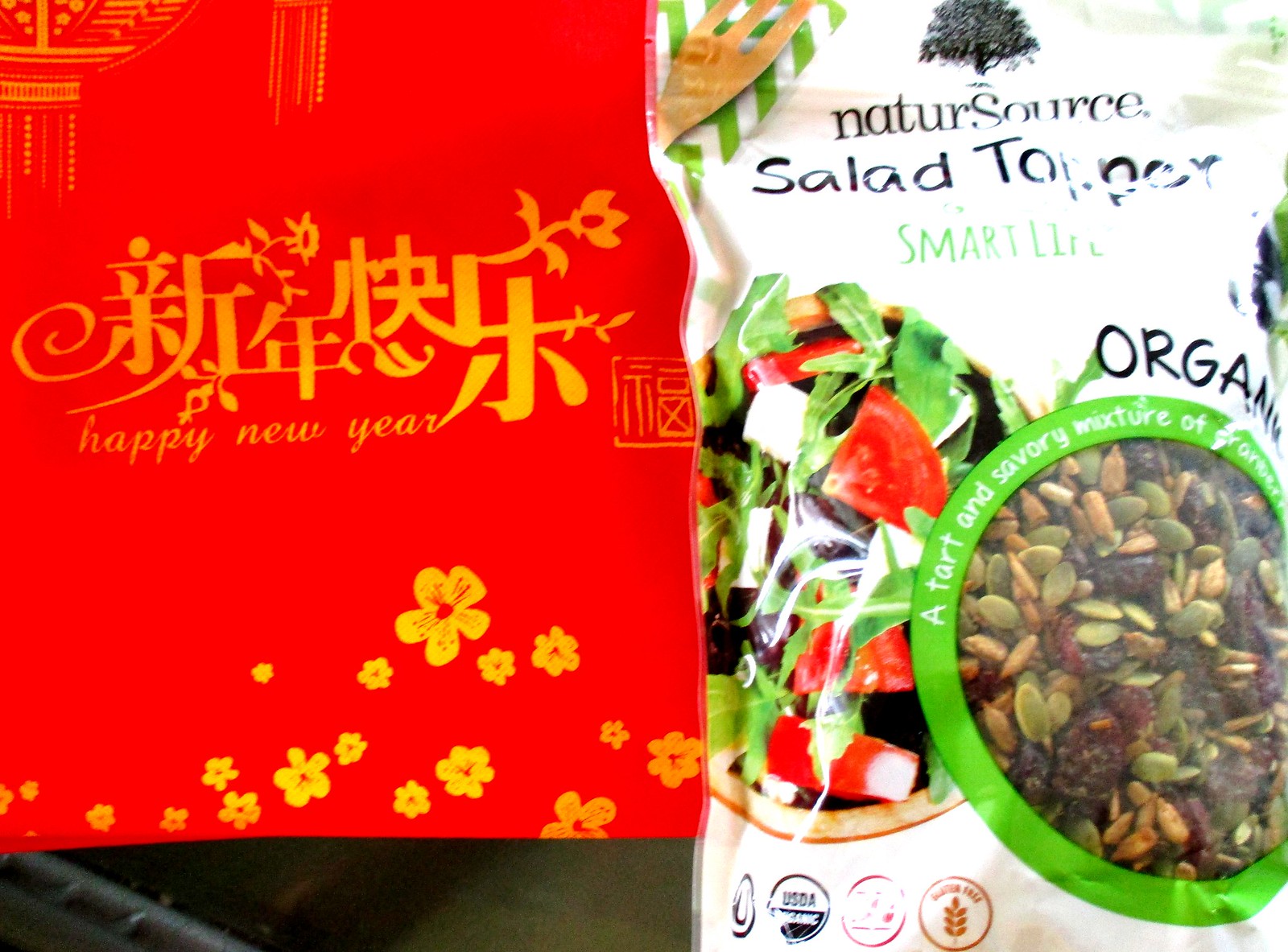The image features a bag of Nature Source Salad Topper prominently displayed against a backdrop. The bag itself is green and white, with a distinctive black logo at the top center, depicting a tree. The text "Nature Source Salad Topper" is displayed in bold black lettering. Below the main text, the bag also bears the inscription "Smart Life," although it is somewhat obscured by lighting. The bag highlights its organic nature and a "tart and savory mixture," hinted at by the smaller, harder-to-read text near the product window. This circular window, located on the right corner, reveals a colorful variety of ingredients including pumpkin seeds, sunflower seeds, dried fruit, and other seeds in green, black, and yellowish-brown hues. 

In addition to the bag, the left side of the image depicts a red piece of paper with gold floral designs and the text "Happy New Year" in yellow and gold script. This paper seems to be part of a box that features Asian-style text and design elements, including a small shrine illustrated at the top left corner and yellow flowers adorning the bottom. The paper's vibrant red color and festive text contribute to a celebratory New Year theme in the overall picture.